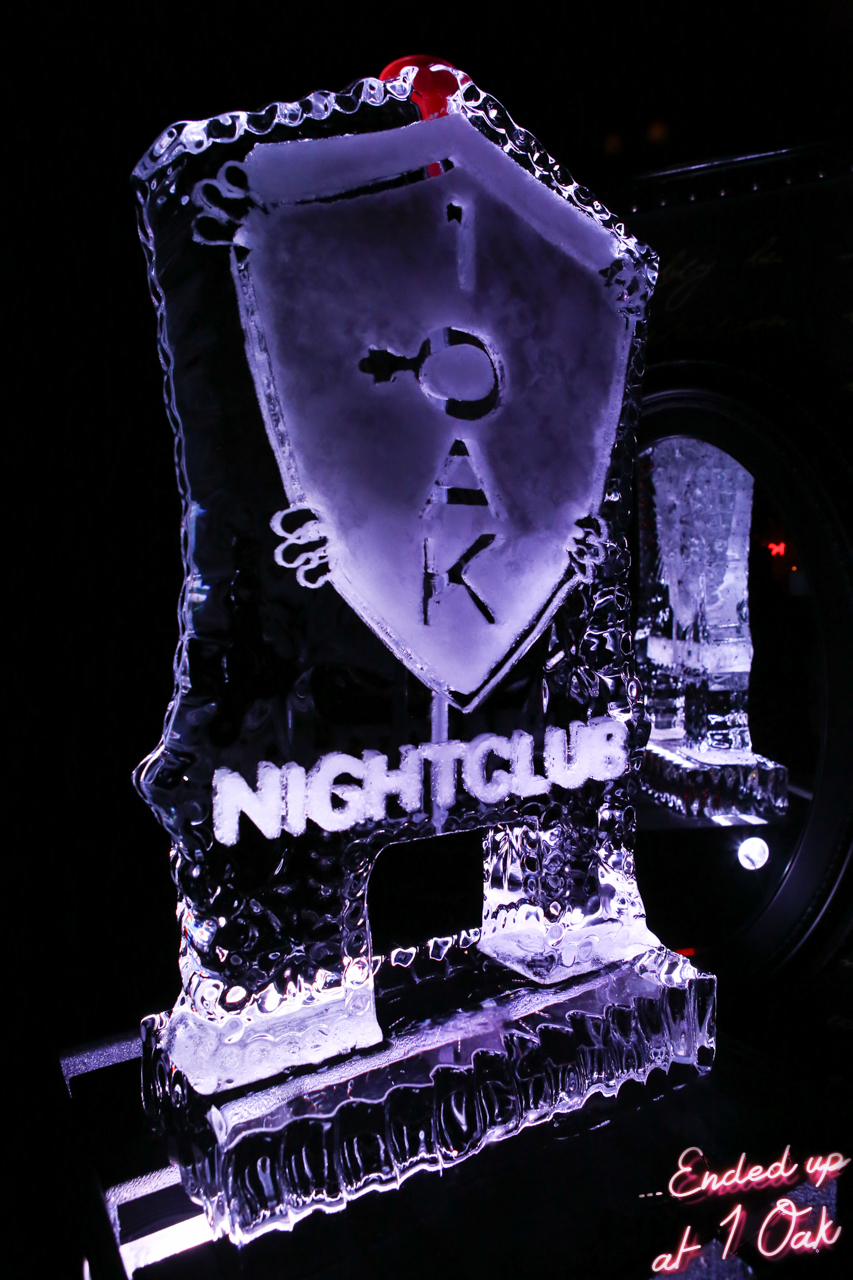In a dimly lit nightclub setting, the photograph captures a prominent large, rectangular ice sculpture at the forefront. The sculpture is mostly transparent, showcasing exquisite craftsmanship with a carved white shield on its front. Inscribed within the shield are the letters and number forming the phrase "One O-A-K" or "One Oak," followed by the word "Nightclub" elegantly etched below. A decorative base supports the intricate design. 

In the background, another identical ice sculpture is positioned, facing in the opposite direction. The image bears a red cursive watermark in the bottom right corner that reads "ended up at One Oak." Further highlighting the nightclub ambiance, a distant small red light is visible next to an oval-shaped mirror, reflecting the back of the ice sculpture. Red lights scatter subtly throughout the room, adding to the atmospheric darkness punctuated only by the glowing details of the sculptures.